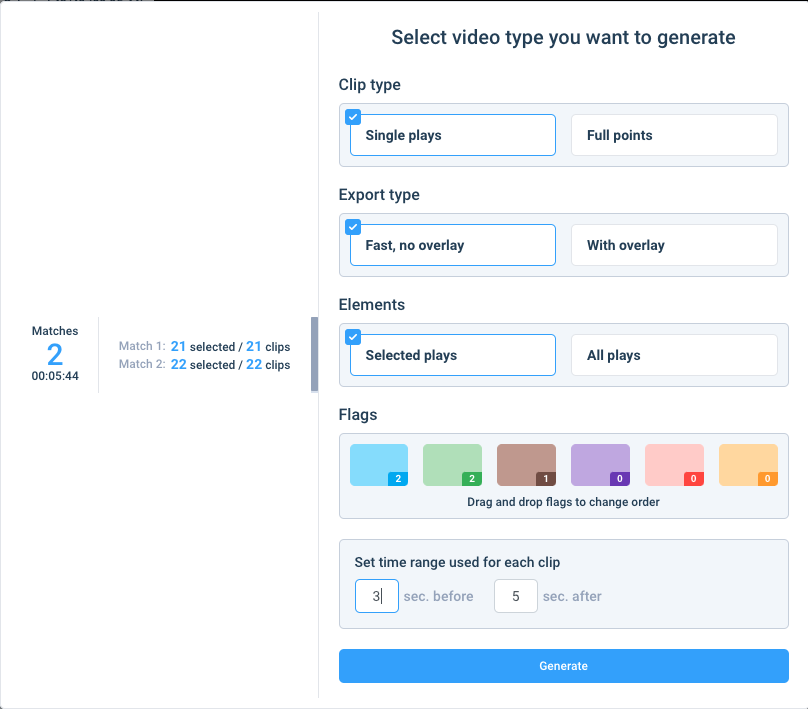Screenshot depicting a user interface for generating video content. The interface is framed by a black bar at the top and gray bars on the left and bottom sides, leaving the right side open. On the left, the section titled "Matches" features a blue number "2" indicator and a timestamp "00:05:44." Below, it lists two matches: "Match 1" with "21 selected out of 21 clips" and "Match 2" with "22 selected out of 22 clips."

On the right side, the interface guides the user to "Select video type you want to generate." Below, the "Clip type" section displays options within a gray bar: "Single Plays" highlighted in white with a blue border, followed by "Full Points." Under the "Export type" section, options "Fast, no overlay" (highlighted with a blue border) and "With overlay" are present. Further down, in the "Elements" section, options "Selected Plays" and "All Plays" are listed with "Selected Plays" chosen.

At the bottom, the "Flags" section features a variety of colored rectangles labeled with numbers: a blue rectangle with "2," a green rectangle with "2," a brown rectangle with "1," and purple, red, and orange rectangles each with "0." A note indicates that users can drag and drop flags to change their color.